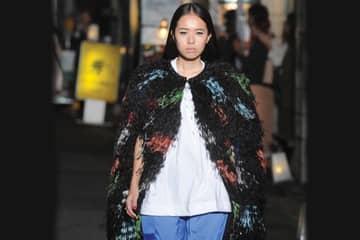The photograph captures a fashion model of Asian descent, showcasing her from the waist up in a rectangular frame with the top and bottom sides twice as long as the left and right sides. The model exhibits a stoic expression and has long, black hair parted down the middle. She is attired in blue silk-like pants, a loose-fitting white blouse, and a distinctive black, feather-like shawl with blue, green, and orange spots, fastened with a clasp at the collar. She appears to be walking confidently towards the front of the image, likely participating in a high-profile fashion show. The focus remains sharply on the model, while the background is blurred, revealing indistinct figures and a white sign. Black borders frame the left and right sides of the photograph, with only a hint of different background shades visible, maintaining an overall emphasis on the model and her attire.